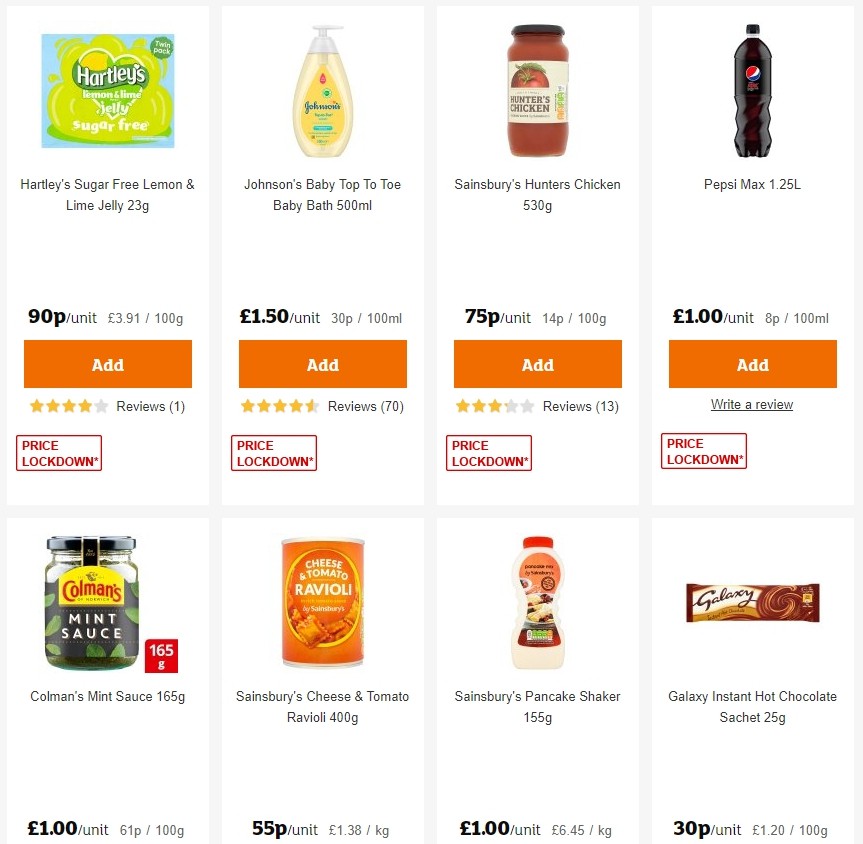This is a detailed screenshot from a generic shopping application, potentially from platforms like Target or Walmart's websites or apps. The design showcases a clean white background, with products displayed in two rows, each row containing four items.

In the top row:
1. **Hartley's Sugar-Free Jelly** - Featuring a blue and green label, priced at 90 pence. Below the product description, there is an orange rectangular "Add" button in white text, consistent with all items in this row. Each product also displays review stars and a "Price Lockdown" tag, indicated by a red outlined white rectangle positioned at the bottom left corner.
2. **Johnson's Baby Top-to-Toe Baby Bath** - Priced at 1 pound 50 pence. Complete with the "Add" button and "Price Lockdown" tag.
3. **Sainsbury's Hunter's Chicken** - Available for 75 pence. Includes both the "Add" button and "Price Lockdown" tag.
4. **Pepsi Max (1.25 liters)** - Priced at 1 pound. This item also features the "Add" button and "Price Lockdown" tag.

In the bottom row, the items do not display the orange "Add" button or the "Price Lockdown" tag, likely because these elements are cut off in the current screenshot. The products are as follows:
1. **Coleman's Mint Sauce** - Priced at 1 pound.
2. **Sainsbury's Cheese and Tomato Ravioli** - Priced at 55 pence.
3. **Sainsbury's Pancake Shaker** - Priced at 1 pound.
4. **Galaxy Instant Hot Chocolate Sachet** - Priced at 30 pence.

The screenshot provides a clear overview of the products available, highlighting key information such as pricing and promotional tags, facilitating easy navigation and selection for the user.